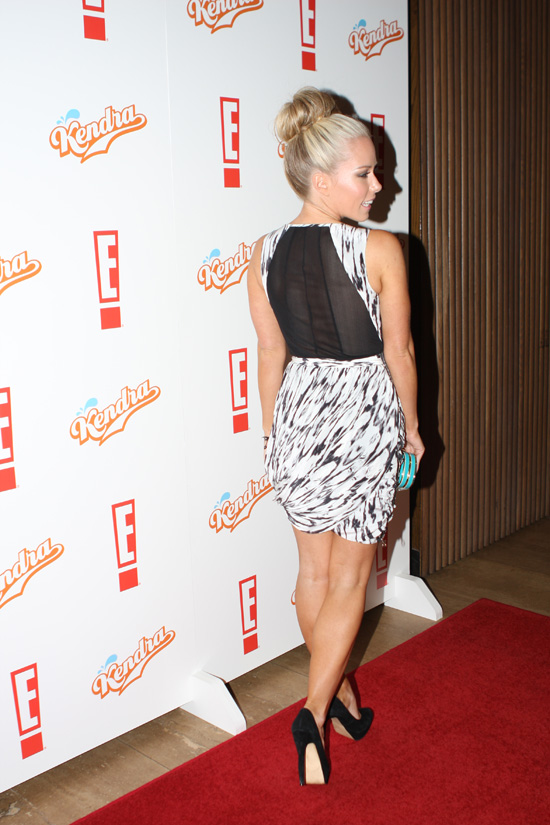The image features a woman, potentially Kendra Wilkinson, standing on a red carpet against a white poster wall. The wall is adorned with repeating logos that feature the name "Kendra" in orange script with an underline, and a red exclamation mark partially covered by a bold, white block letter 'E'. The woman displays a slim build and is of short stature, with her back toward the camera as she looks to her right. Her footwear consists of black high heels, and she appears to be holding a light blue clutch in her right hand. Her dress is a striking black and white zebra pattern, with a sheer black mesh fabric on the back. Her blonde hair is styled up in a bun. The setting is vibrant and well-lit, showcasing colors that range from red to white, orange, black, and blue, all contributing to the detailed and vivid presentation of the scene.